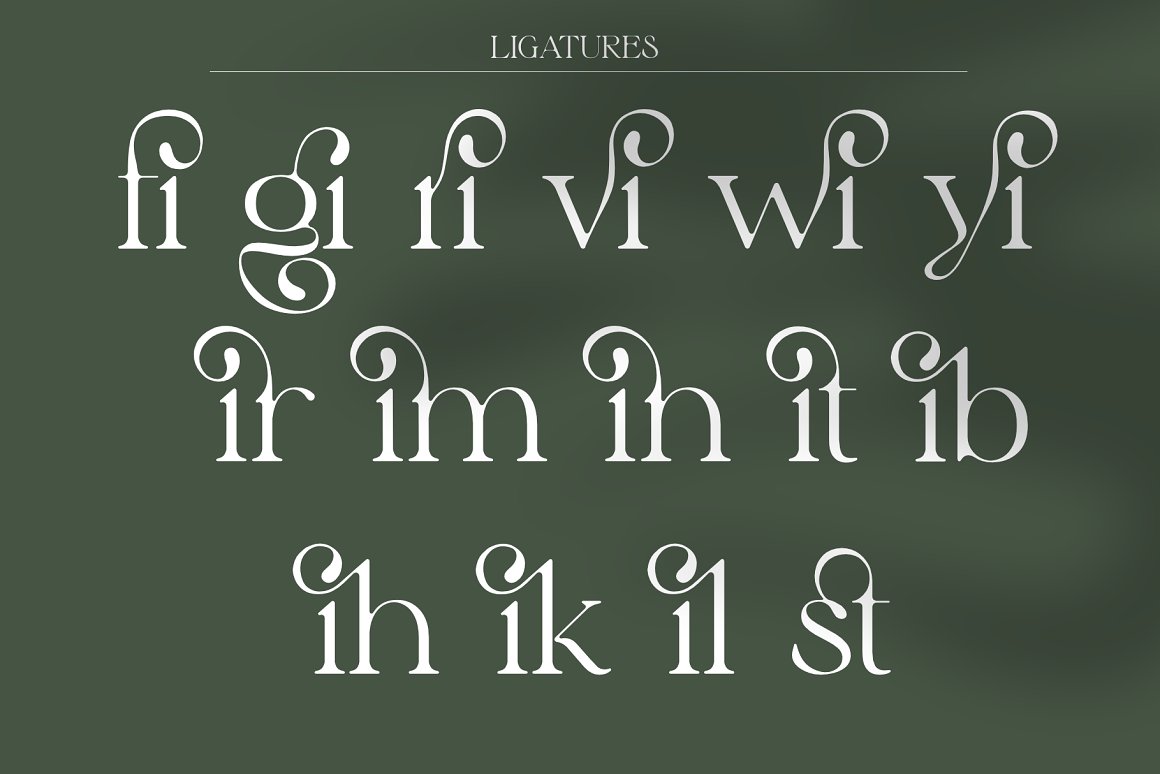The image presents a rectangular poster set against a dark green, slightly mottled background. At the top, in bold white letters, it reads "LIGATURES," which is underlined by a thin white line. Below this heading, the poster showcases examples of ligatures — pairs of letters elegantly combined into unique symbols. The ligatures are organized into three horizontal rows of white text. The first row, containing "fi," "gi," "ri," "vi," "wi," and "yi," is the longest. The second row, slightly shorter, features "ir," "im," "in," "it," and "ib." The third and shortest row includes "ih," "ik," "il," and "st." Each ligature merges the letters with intricate designs and loops, emphasizing the artistic nature of this typographic feature.